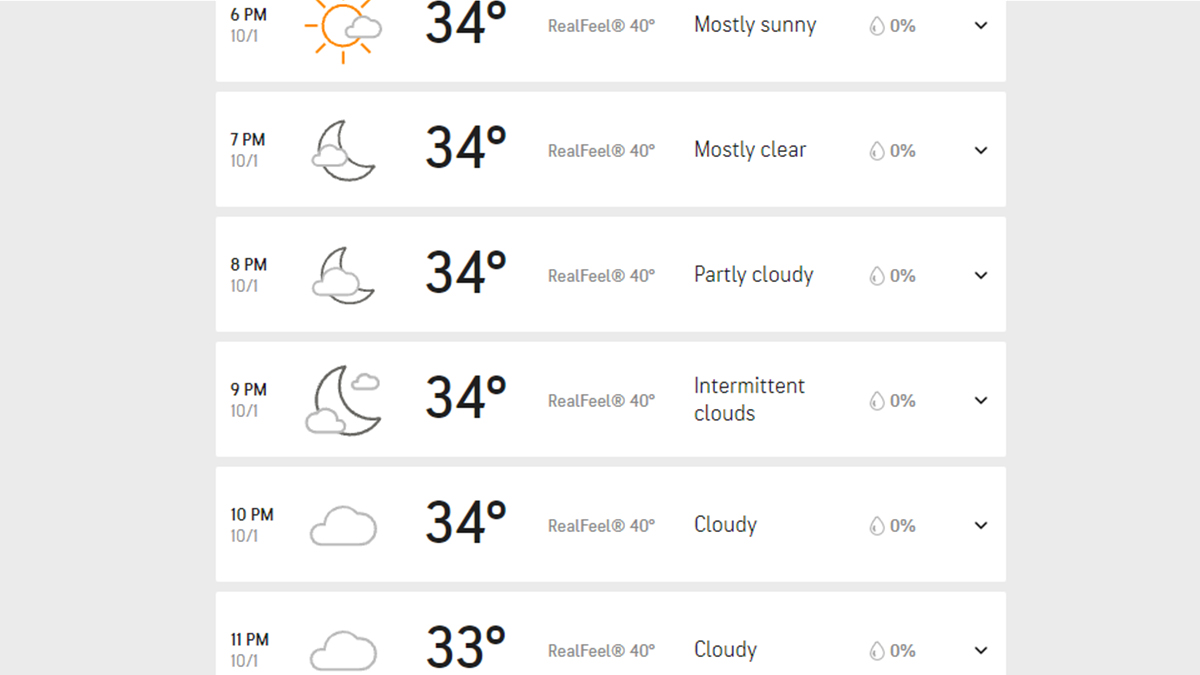Here is the cleaned-up, detailed caption:

---

This image is a screenshot of a weather forecast for October 1st. It provides a detailed hourly breakdown of the weather conditions for that day. 

- **Temperature:** The temperature remains consistent at 34°F throughout the day, dropping slightly to 33°F at 11 p.m. 

- **Weather Conditions:** 
  - From 6 p.m., the weather is mostly sunny with few clouds.
  - At 7 p.m., the sky is mostly clear.
  - At 8 p.m., it transitions to partly cloudy.
  - By 9 p.m., the sky shows intermittent clouds.
  - From 10 p.m. to 11 p.m., it becomes fully cloudy.
  
- **Precipitation:** There is a 0% chance of precipitation throughout the entire day.

- **RealFeel® Temperature:** Despite the actual temperatures, the RealFeel® readings indicate that it will feel like 40°F at every hour listed.

This basic forecast provides a comprehensive look at the weather conditions expected on October 1st, assuring no precipitation and a consistent real-feel temperature despite slight variations in actual temperature.